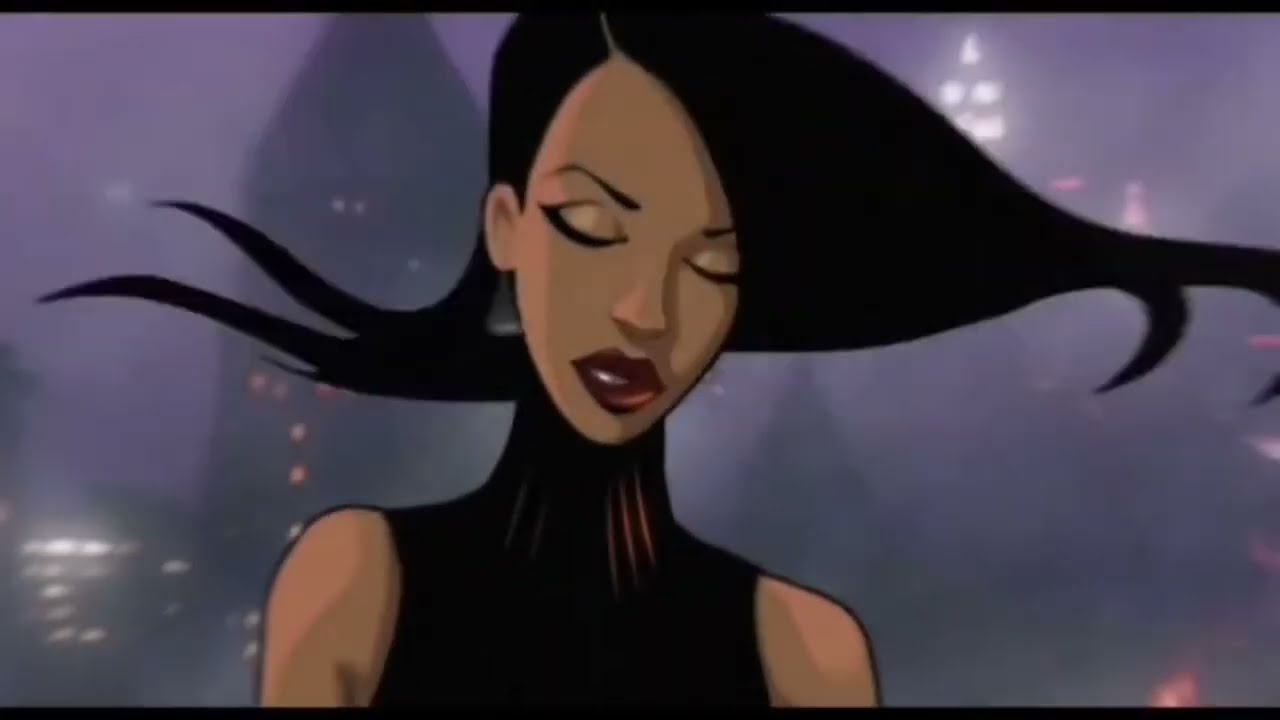The digital image depicts an animated young woman with a caramel skin complexion and long, dark hair blowing in the wind. She is centered in the image, wearing a sleeveless black turtleneck that accentuates her narrow neck. Her eyes are closed, revealing dark eyelashes and eyebrows, with her slightly parted lips adorned with dark red lipstick. The background features a hazy, light purple hue with blurred skyscrapers, one of which is visible over her right shoulder. Scattered lights from the buildings suggest the time is either night or dusk, adding a dreamy atmosphere to the scene. The overall style and detailing suggest that this image could belong to a digital artwork or a video game, characterized by its cartoon-like quality.